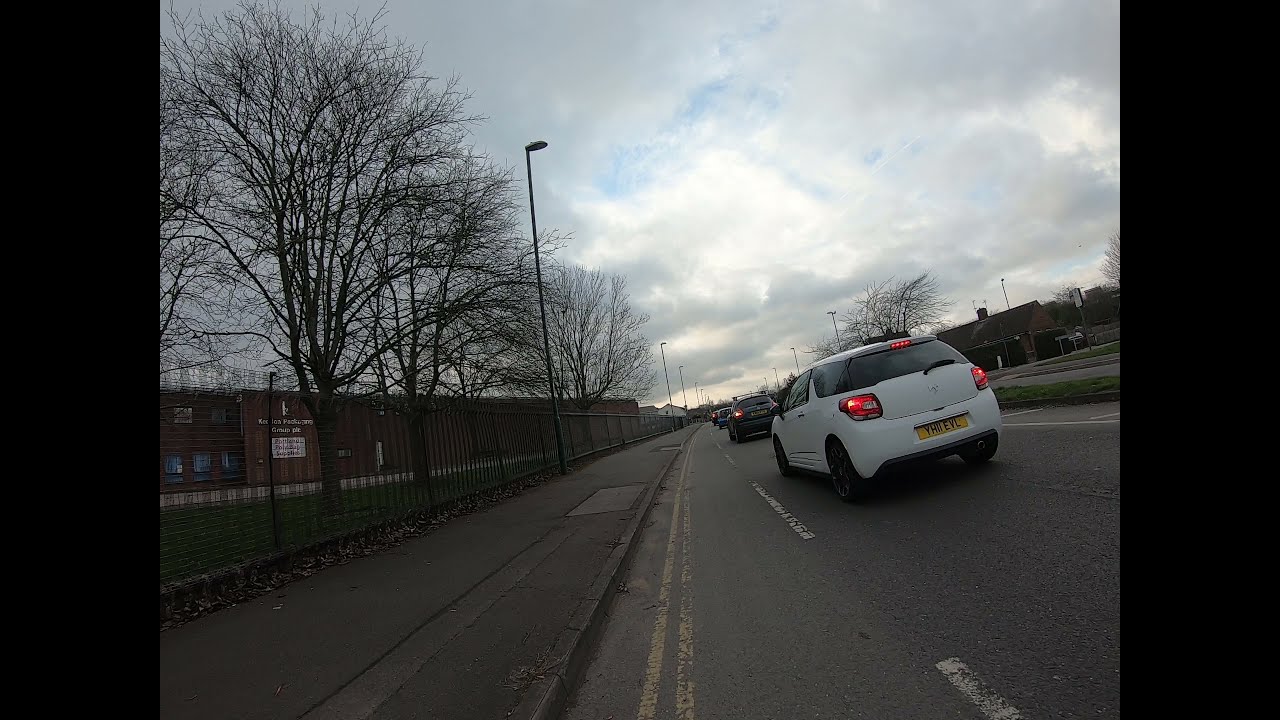This detailed landscape orientation image, possibly a GoPro video freeze-frame, captures a cloudy day scene along a highway road just right of the sidewalk. The vantage point is from the bike lane on the left side of a line of cars, with a white hatchback, possibly a Nissan, as the closest vehicle, its brake lights glowing red. The blue lettering on its license plate reads YHQEYL. Ahead of it are more vehicles, waiting possibly to pick up kids from a nearby school. 

To the right of the road, there's a house, while on the left, a giant building, presumably a school, stands behind a long line of see-through black fencing. A white logo on the building's front is unreadable from this distance, and bare trees are scattered within the fenced area. A large streetlight is visible on the sidewalk near these trees. There is a grass-covered median dividing the lanes. Further to the left, there is a concrete area with a floodlight and more leafless trees, emphasizing the season's bleakness. 

The scene is cast in low light due to the extremely cloudy sky, with a mix of white and gray clouds suggesting either late afternoon or early evening. A small brown building with a black roof and a sign is also seen on the right side, possibly a business. The overall image is dark and moody, highlighting the realism and detailed representational style of the photograph.